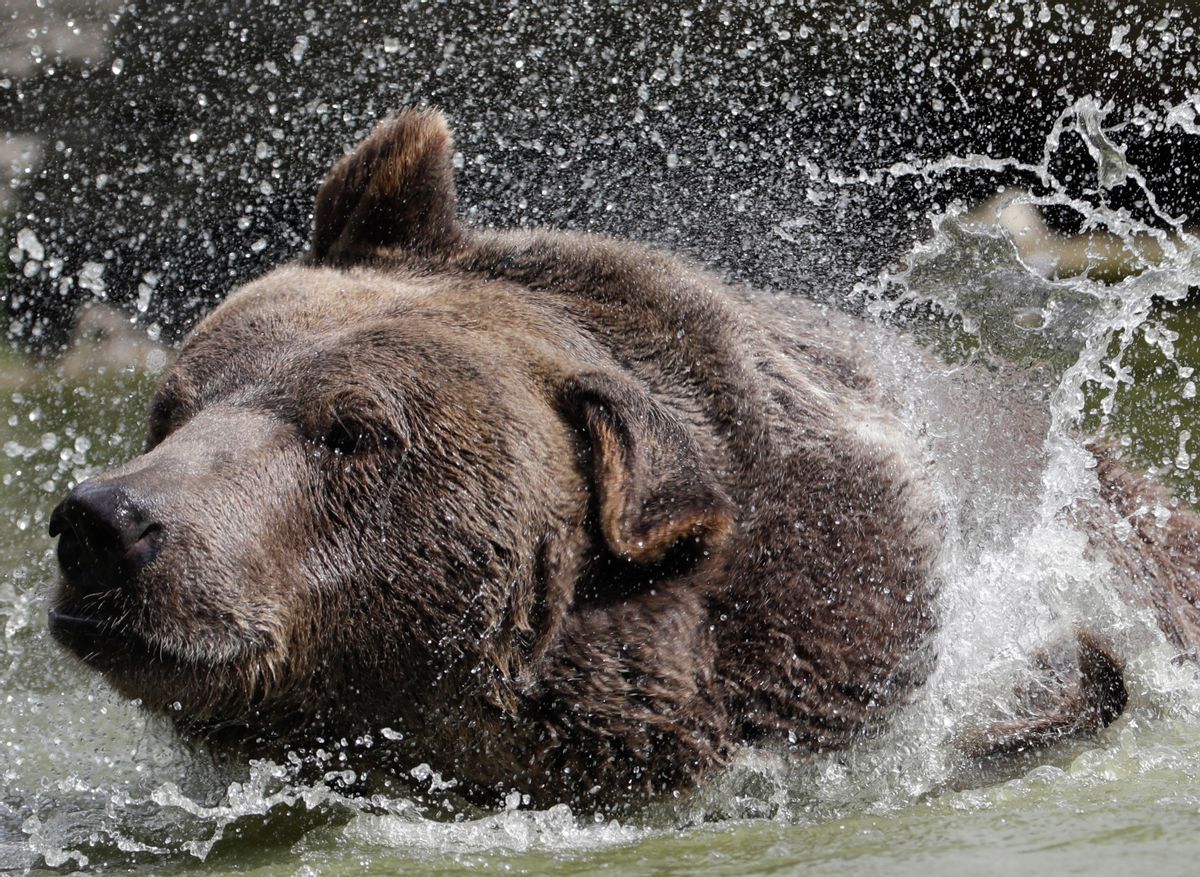The photograph captures the dramatic moment of a dark brown bear, likely a grizzly, either emerging from or plunging into a body of greenish-brown water. Most of the bear's body is obscured by a large splash on the right-hand side, with water droplets filling the air, creating an almost misty effect that conceals any background details. We see the bear at a roughly 45-degree angle, with its head and part of its back visible above the water's surface. The bear's right ear is perked up while its left ear flops down. The bear's wet fur clings to its head, accentuating its black nose and dark eyes, which are looking off to the left side of the frame. The close-up shot, seemingly taken with a high-speed shutter, freezes the dynamic splashes and droplets around the bear, sharply focusing on the animal amidst the chaotic water.